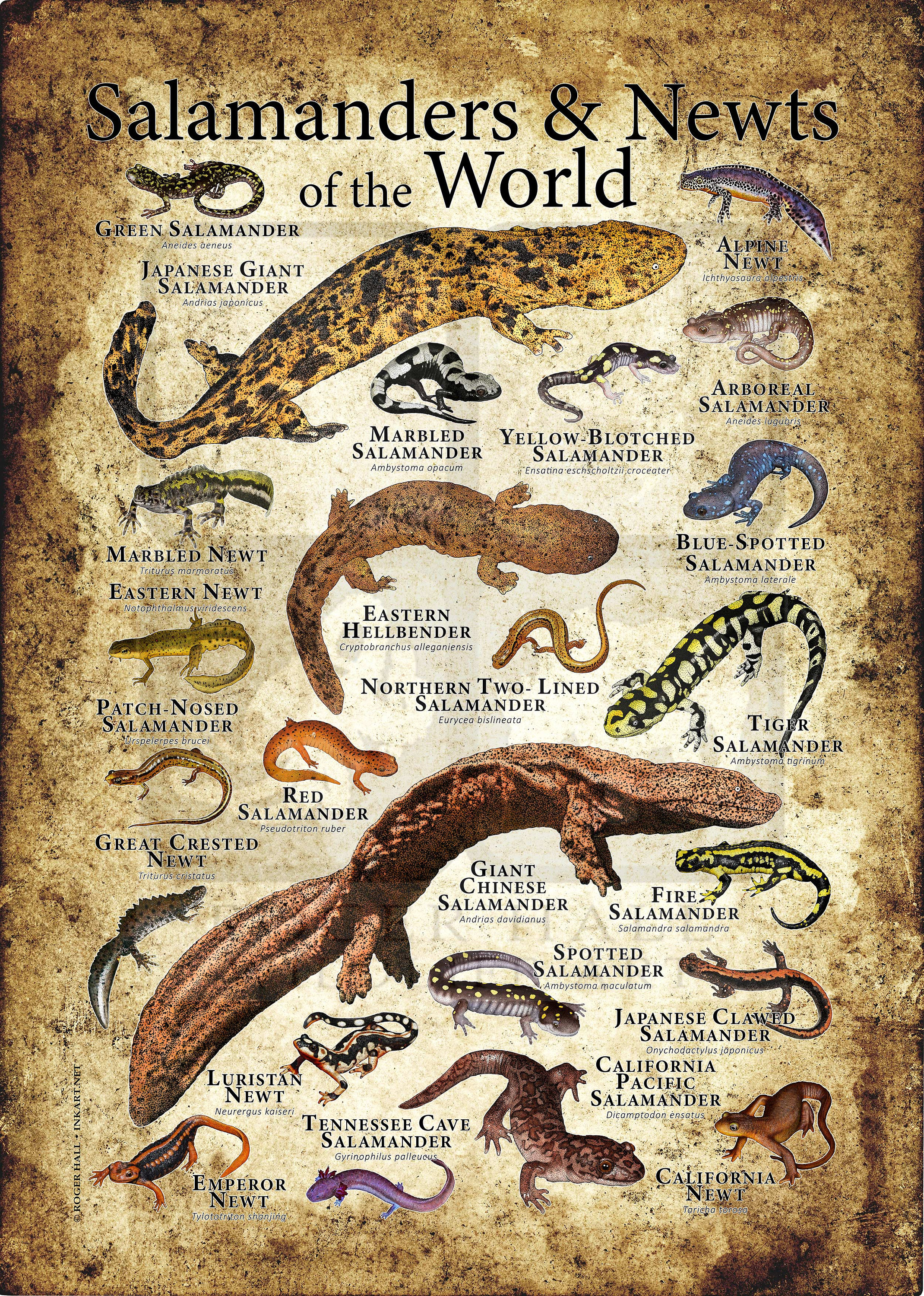This vertically aligned rectangular poster or sign showcases an array of "Salamanders and Newts of the World," as stated in bold, black text centered at the top. The background features shades of brown, transitioning from a medium speckled brown along the edges to a tan or beige center, along with a dust effect that gives it a rustic appearance. The poster is adorned with detailed illustrations of approximately 20 different salamanders and newts, each meticulously labeled with their respective names.

In the upper left corner, the "Green Salamander" is depicted, followed by the "Japanese Giant Salamander." The upper right hosts the "Alpine Newt" above the "Arboreal Salamander." Below these, a large spotted salamander grabs attention. Central figures include the "Eastern Hellbender," "Northern Two-Lined Salamander," and the prominently large "Giant Chinese Salamander," surrounded by smaller varieties. Among the diverse palette, there are vibrant colored species such as the yellow and black "Fire Salamander" and the completely red "Red Salamander."

The salamanders and newts are illustrated in a spectrum of colors ranging from browns and blacks to oranges and purples, each highlighting their unique shapes and sizes. This visually rich and well-labeled compilation offers a comprehensive depiction of these captivating amphibians.